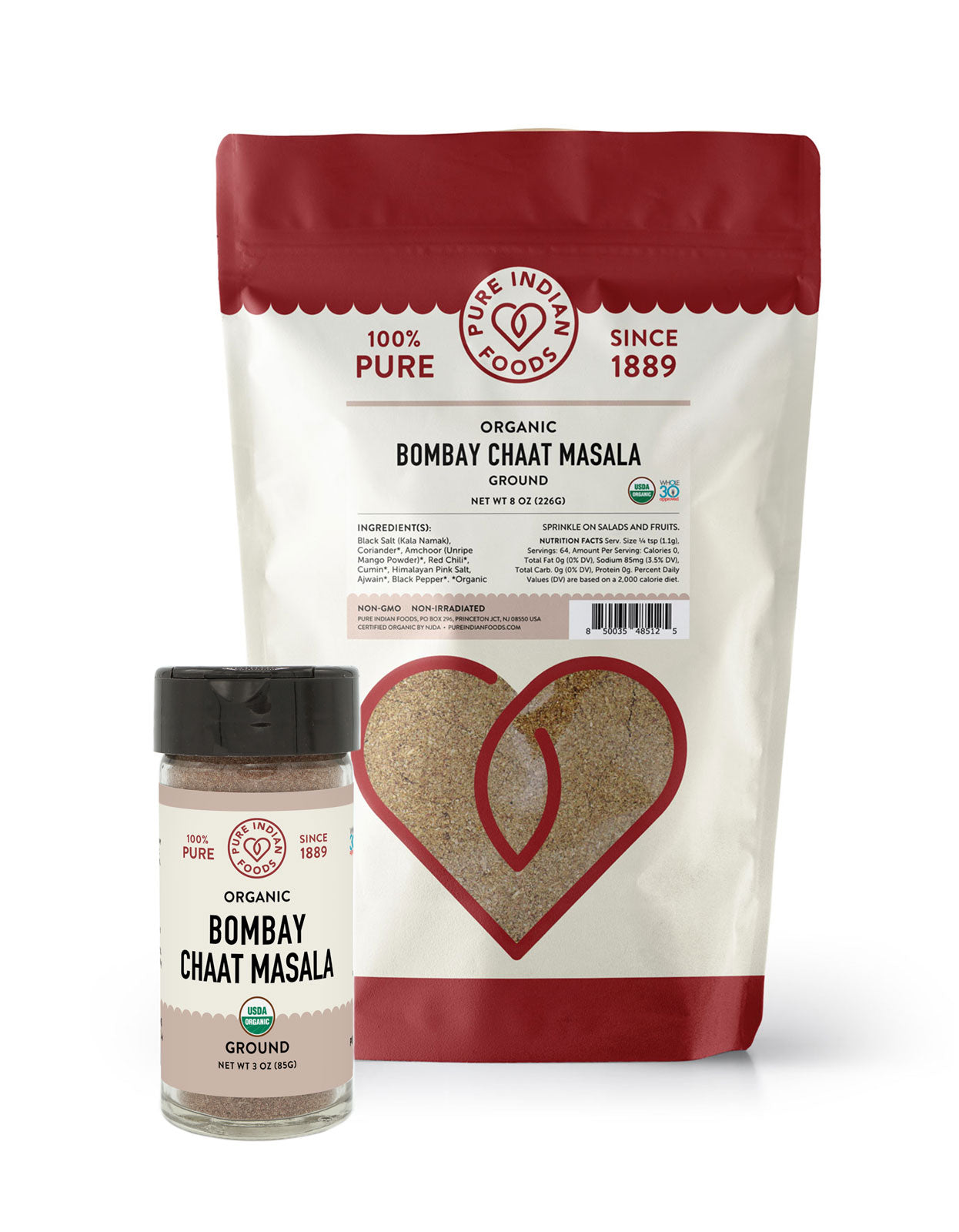The image features a package and a small bottle of organic Bombay Chat Masala from Pure Indian Foods, a brand renowned for its 100% pure products since 1889. The primary package is an 8-ounce plastic pouch with a dark red-maroon border at the top and bottom, which features a curved half-circle design. Between these borders, the pouch is tan-colored and includes a clear heart-shaped window through which the light brown, ground seasoning is visible. The red font prominently displays "100% pure" along with the Pure Indian Foods logo containing a red heart, and the text "since 1889." Below this in smaller black font, it reads "organic Bombay chat masala, ground," along with the net weight of 8 ounces. The ingredients list, due to its small size, is difficult to read. In front of the pouch, a smaller cylindrical glass bottle with a black cap displays the same details: "organic Bombay chat masala, ground," with a clear body allowing a view of the spice inside. The packaging emphasizes the non-GMO and non-irradiated nature of the spice mix, suggesting it is perfect for sprinkling on salads and fruits.